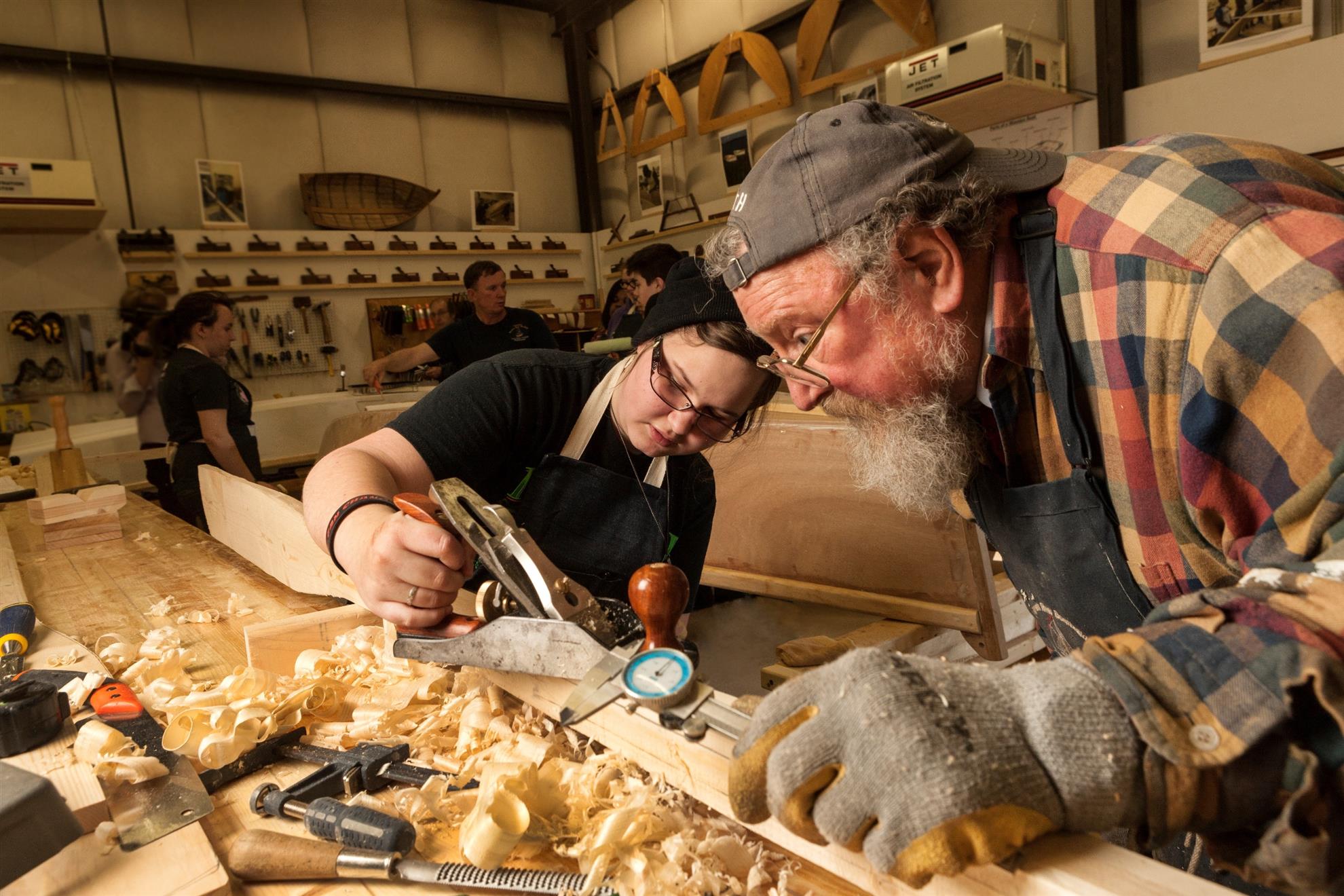In a cozy, wooden-paneled workshop with off-white walls adorned with various trinkets and woodworking tools, a detailed scene unfolds. In the foreground, a young woman wearing glasses and a black shirt stands at a workbench covered in wood shavings and tools. She is intently focused on a woodworking project, holding a tool designed for either shaving or measuring. Beside her stands an older man with a gray beard, also wearing glasses, a flannel shirt, gray gloves, and a backward gray ball cap. He holds a tool with a blue gauge and appears to be guiding her. Scattered around them on the workbench are various woodworking instruments and carvings. In the background, two or three more individuals can be seen, adding to the bustling yet focused ambiance of this finely detailed woodworking space.